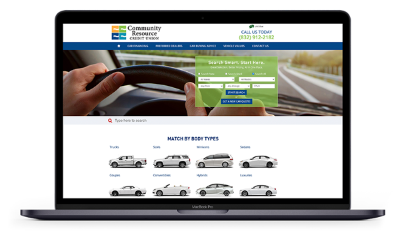The image displays a laptop screen showcasing a website. The website header prominently features the phrase "Community Resource" in black text set against a white banner extending horizontally across the screen. Positioned next to this banner is a multicolored box—comprising shades of green, orange, blue, and light blue—that highlights the message "Call us today" alongside a provided 800 number. Below these elements, a blue horizontal bar spans the width of the screen.

The central part of the website contains an image depicting a person driving a car, as seen from behind. The driver’s hands are visible on the steering wheel, and the view extends through the windshield, showing the road ahead complete with white lane markings and roadside trees on the right.

In the foreground of this scene, a green pop-up box appears, featuring multiple white input fields presumably for user information. Below these fields are two blue buttons.

Further down in the website's body, there is a small red sign with black text. The main content area provides information on matching cars by body type, displaying various car models all colored in white. Each car is accompanied by a label positioned to the upper left of the respective vehicle's image.

Together, these elements give a comprehensive visual and functional overview of the website's offerings.